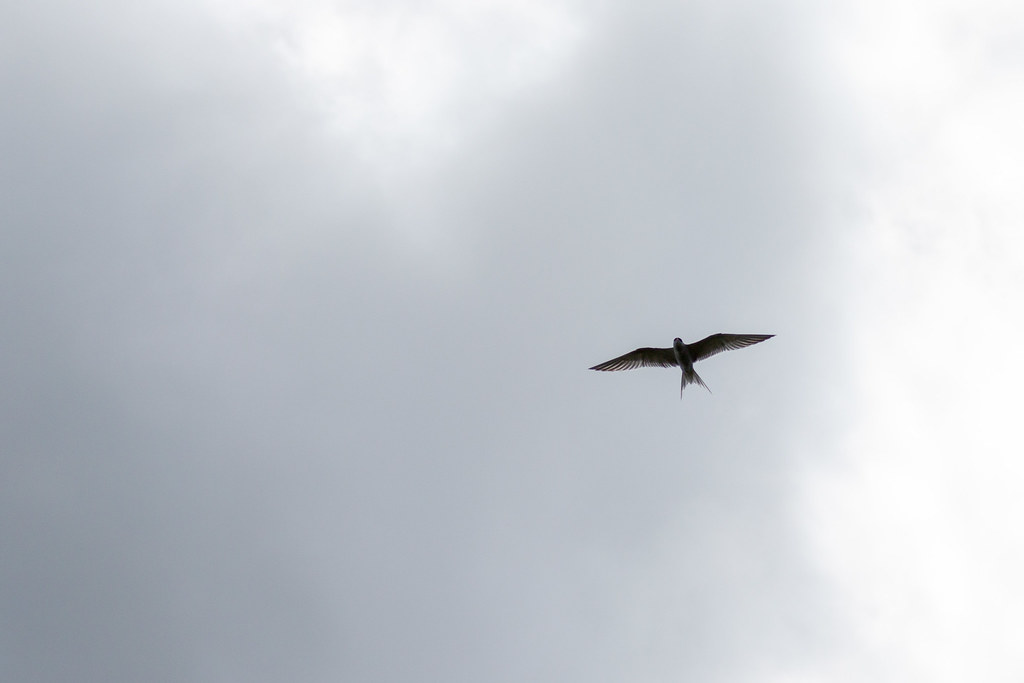In this horizontally aligned, rectangular outdoor image taken during the daytime under a very cloudy sky, the scene is dominated by varying shades of gray clouds with a few areas of lighter, almost white clouds. There's a small section where the clouds are less dense, allowing a hint of sunlight to peak through. At the right-hand side of the image, towards the middle, a large black bird is showcased as it glides effortlessly with its wings fully spread. The perspective appears to be from beneath the bird, capturing its underside as it soars. The bird seems to be predominantly black, with possible hints of gray on its tail. The overall atmosphere depicted is one of overcast skies, with the bird seemingly floating prominently against the muted backdrop.